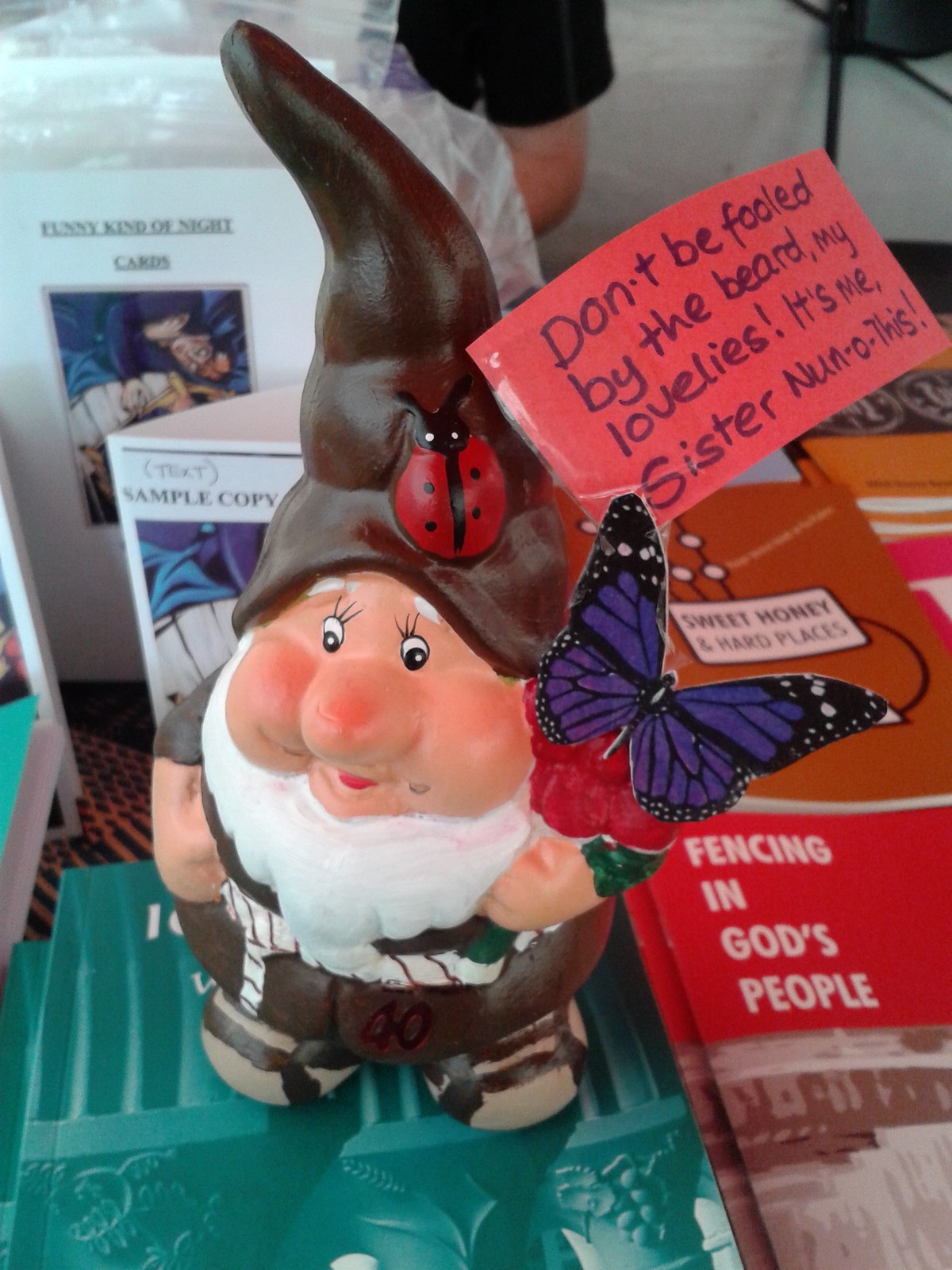On a cluttered table or shelf, the focal point is a charming gnome-like figure with chubby cheeks and a fluffy white beard. The gnome wears brown pants and a long, cone-shaped brown hat decorated with a ladybug. On his left shoulder rests a purple butterfly. A tag attached to the gnome, with red and black lettering, reads, "Don't be fooled by my beard, my lovelies. It's me, sister none of this."

Surrounding the gnome are various pamphlets, magazines, and cards. One card prominently displays a cartoon picture with the title "Funny Kind of Night Cards," while another one labeled "Text Sample Copy" stands next to it. In the lower corner, a magazine with a red top half featuring white lettering reads "Fencing and God's People." The gnome seems to be standing on some paper with a green-colored image. Additionally, a brown-colored image with black letters spells out "Sweet Honey and Hard Places."

In the background, a person's left arm, clad in a short-sleeved black shirt, is faintly visible, adding a human element to the scene. The overall color palette in the image includes shades of purple, pink, white, brown, green, and red, contributing to a lively and whimsical atmosphere.